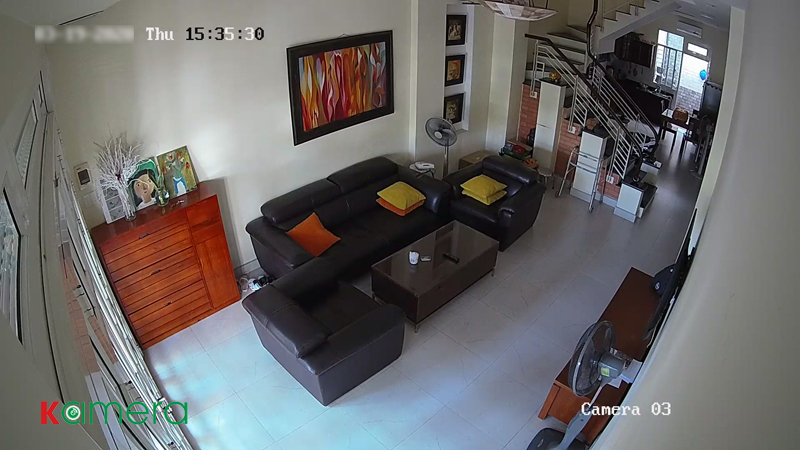This photograph, likely captured from a security camera mounted in the top left corner of a room, provides a comprehensive view of an elegantly furnished interior. The timestamp, although slightly blurred, indicates the image was taken on a Thursday at 15:35:30. Bold, red text with a green outline reading "K AMER A" appears in the bottom left corner, while "CAMERA 03" is displayed in white text about two inches to the right.

From the bottom left corner, a small section of a wall ascends upwards, featuring two windows and a glass door adjacent to it. To the right of this glass section, a white wall extends, ending at a corner where a brown desk is positioned. Dominating the central part of the room is a black couch flanked by black chairs on either side. In front of this setup, a glass-topped table is neatly placed on the white marble or hardwood floor. 

A visually striking painting composed of various colors with a black border is hung above the couch. The couch is also accented with bright yellow and red pillows at each end. Moving rightward, there is a staircase ascending from the right to the left, then turning upwards out of the camera's frame, featuring black railings and white sides.

Above the couch area, a ceiling fan and a light fixture can be observed. In the far distance beyond the staircase, a second glass door is visible. The right-hand side of the room includes a white wall with the upper portion of a wooden desk and a standing oscillating fan placed near its base. This detailed arrangement reveals a thoughtfully designed and well-maintained living space.